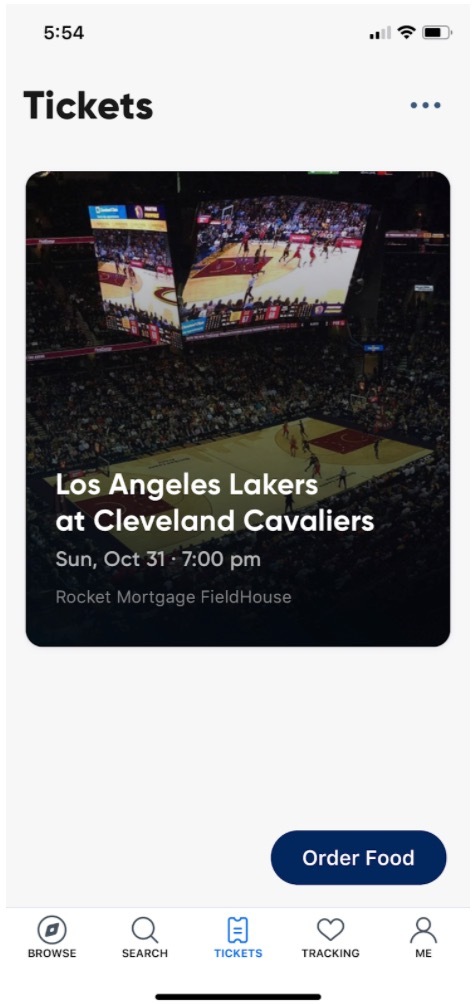This screenshot displays the current time as 5:54 without specifying AM or PM. At the top left corner, the word "Tickets" is prominently shown in bold black font. Below, there is an image of the Cleveland Stadium featuring jumbo screens positioned above the basketball court, providing a central focus. The court is surrounded by a full house of fans, indicating a well-attended game. The text detailing the event reads "Los Angeles Lakers at Cleveland Cavaliers, Sunday, October 31st at 7 PM, Rocket Mortgage Fieldhouse." This information is directly related to the image. At the bottom of the screen, there is a navy blue pill-shaped button labeled "Order Food." Further down, the menu options—"Browse," "Search," "Tickets," "Tracking," and "Me"—are listed. The "Tickets" option is highlighted in bright blue, confirming that this screen is currently active.